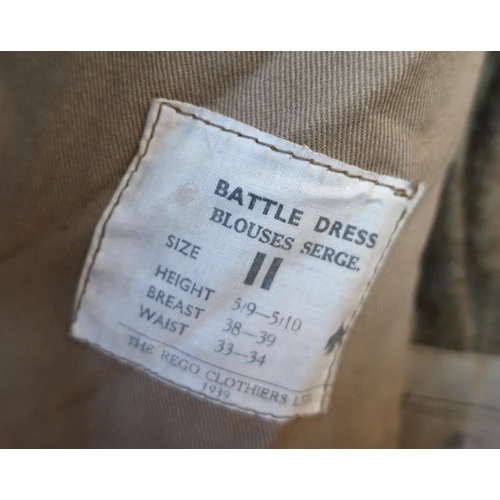The image showcases a zoomed-in view of a white tag stitched onto a medium brown, potentially denim-like, garment. The tag, bordered by dark brown stitching, contains text in dark gray or black. It reads "Battle Dress Blouse's Surge" along with detailed size information such as "Size 11" and measurements for height (5'9" to 5'10"), breast (38"-39"), and waist (33"-34"). Below this information, separated by a horizontal divider, is the manufacturer’s name: "The Rigo Clothiers Limited, 1939." The garment, which could be a blouse or dress, has a discernible pattern and texture, highlighted by the close-up nature of the image. Some wear and smudges are visible on the tag, indicating the garment's use. The backdrop of the image includes a slightly lighter floor adjacent to a darker wall, adding depth to the composition.